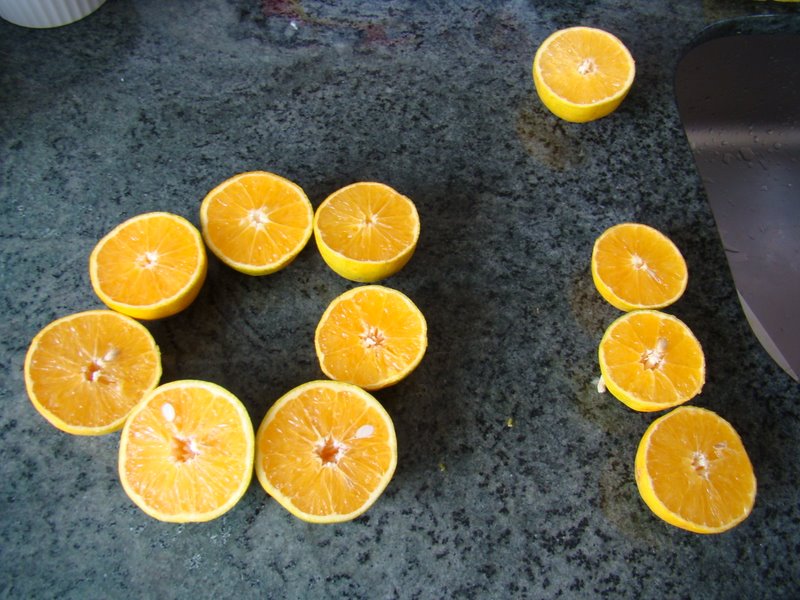This is a detailed color photograph depicting an arrangement of sliced oranges on a dark gray and black speckled granite countertop. The camera angle is from above, capturing the vibrant, bright orange interiors of the seven orange halves arranged in a tight circle, all touching each other. Notably, some of these halves display small seeds near their centers. These orange slices, which have a yellowish tint on the outer peel, measure about three to four inches in diameter, confirming they are oranges. To the upper right of this arrangement, an additional orange half sits alone, while three more orange slices, stacked vertically, can be seen just below this lone piece. The countertop features a slight curve on the right side leading toward a stainless steel sink, around which small drops of water are visible. In the periphery, a silver object is partly visible to the right, and a white ridged container or object can be spotted in the upper left-hand corner of the frame.